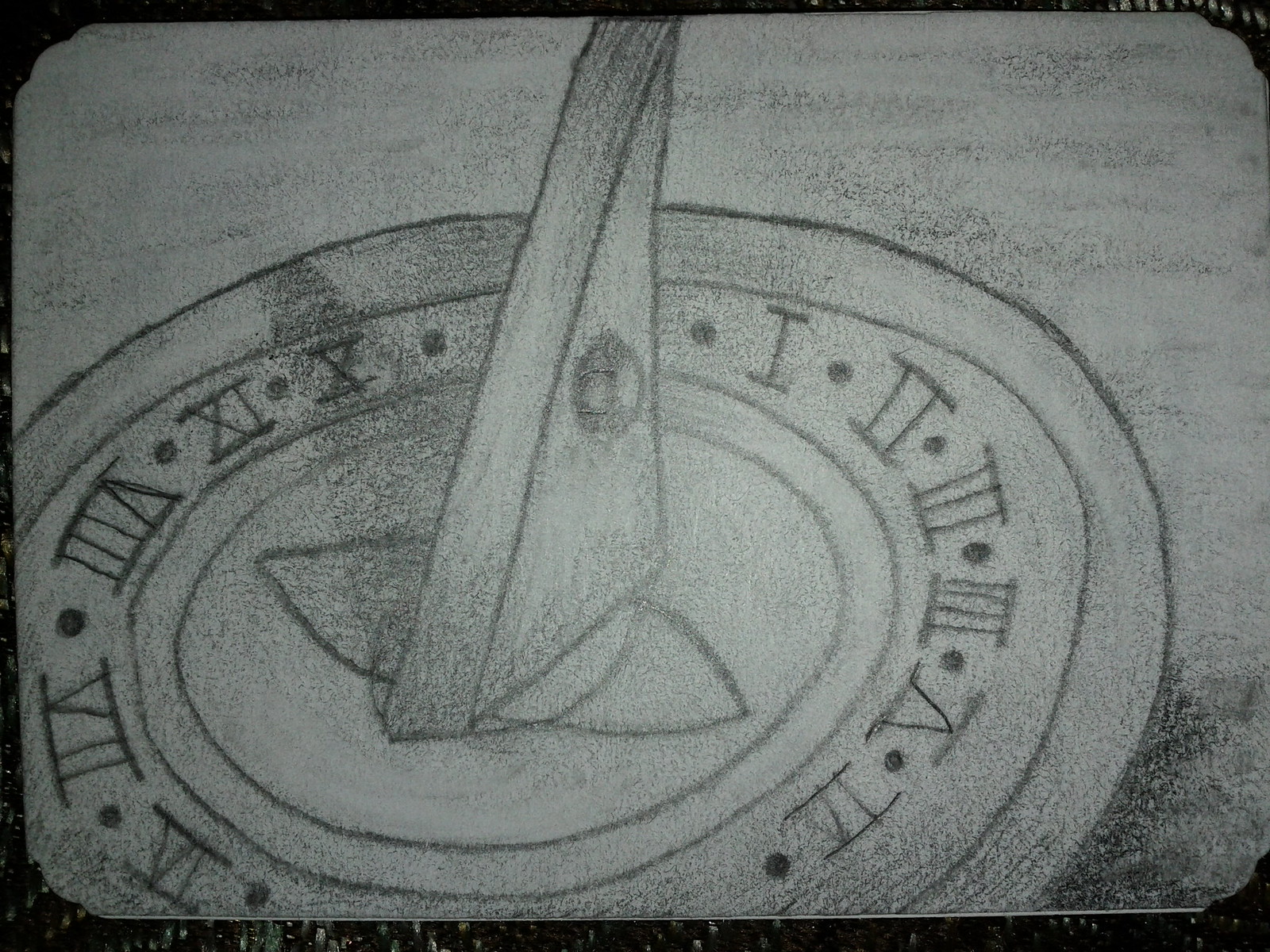This detailed depiction showcases a close-up view of a pencil or charcoal drawing of a sundial meticulously sketched on an undefined surface. The sketch features a series of four concentric circles radiating from the central element of the sundial — a prominent triangular fin or pointer. Encircling this fin on the third ring are carefully drawn Roman numerals, each separated by a small circular mark. The fin casts a distinctive shadow over the numeral X, adding depth and realism to the artwork. In addition to the pointer, two pointed leaf or flower petal shapes are sketched beneath it, adding to the intricate details of the piece. The drawing is filled in with light gray shading throughout, ensuring no part of the surface remains stark white, achieving a consistent texture that subtly emphasizes the details. The image appears to occupy approximately three-quarters of the square canvas and is partially framed in black at the bottom, which suggests a formal presentation.